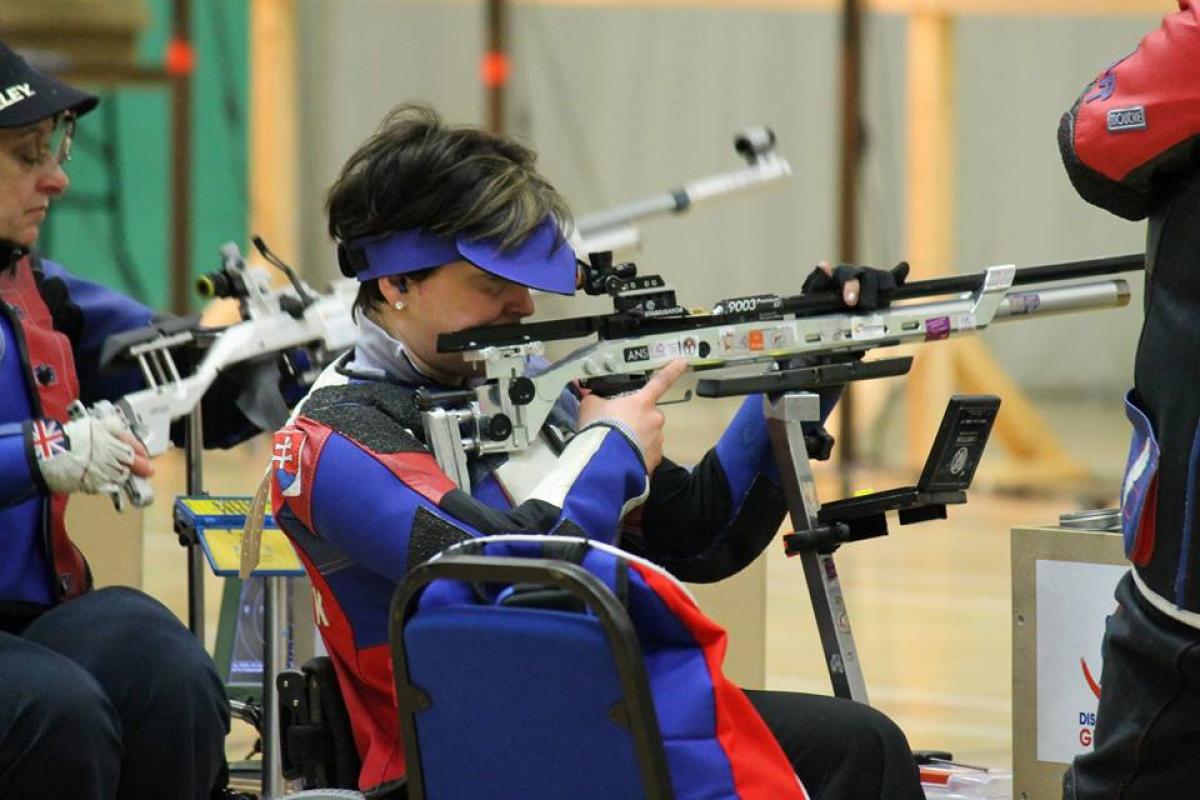In this indoor image, possibly taken in a gymnasium with a wooden or laminate floor, we see two women positioned centrally to the left. Both women are participating in a shooting competition, clad in uniforms predominantly featuring red, blue, black, and white colors. They each wear caps with a prominent brim; one woman's cap is blue, and the other’s is red. The woman in front is aiming a grayish metallic gun with a black top, supported by a stand, while the other woman behind her is similarly equipped but distinguishable by her white gloves compared to the front woman's black glove. Both appear focused, gazing through the sights of their firearms. In the right background, a figure in a black or blue tracksuit with red accents, likely an instructor given his uniformed appearance, observes the scene. The blurred walls in the background appear gray and green, with glimpses of some yellow metal poles, possibly support beams, adding to the indoor ambiance.